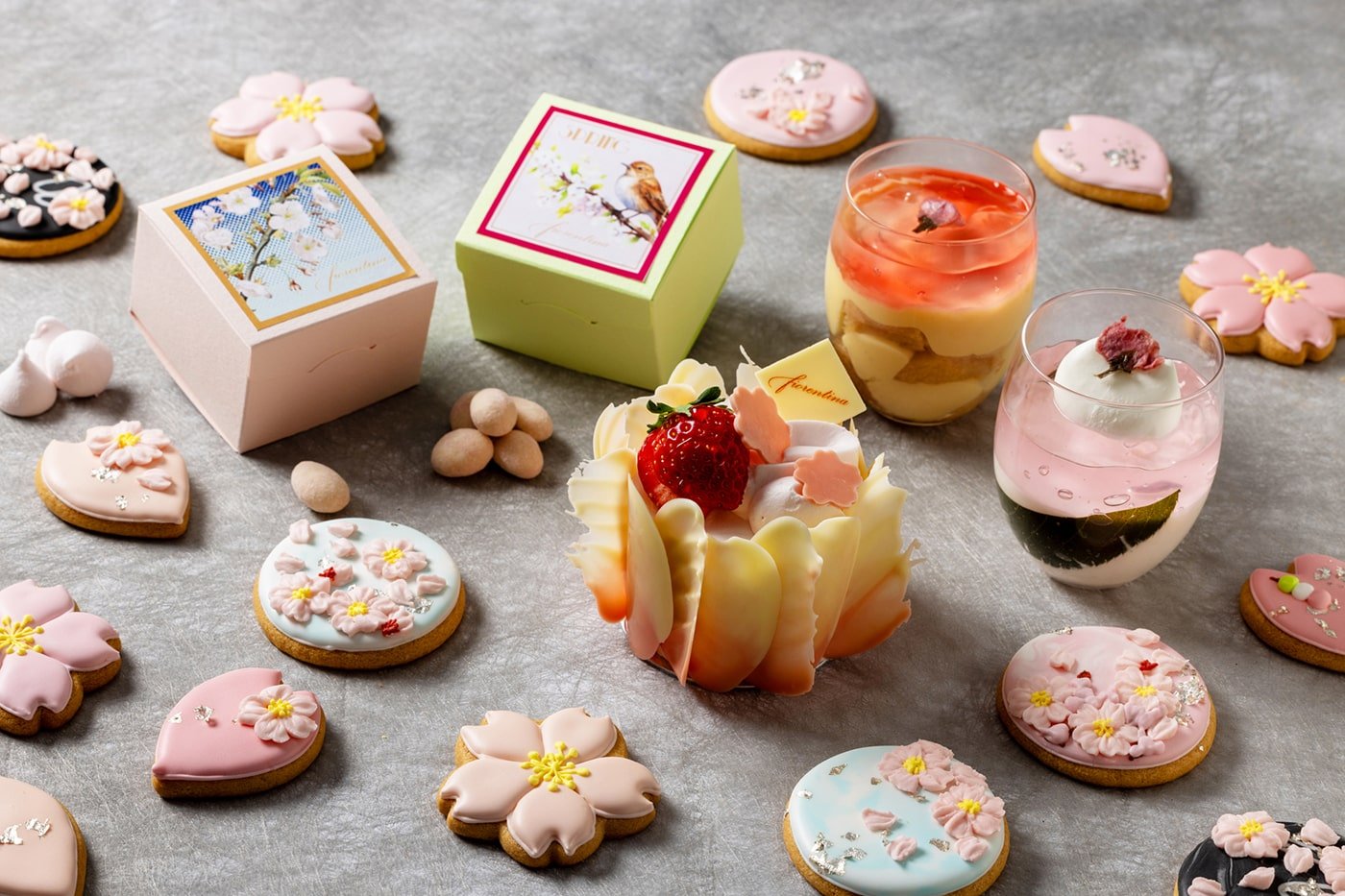The image showcases an assortment of vibrant, spring-themed desserts arranged on a marble surface. The spread prominently features a wide variety of pink and blue cookies, many adorned with intricate cream and floral designs. At the center is a notable pastry, elegantly decorated with chocolate leaves and topped with a fresh strawberry. Accompanying the cookies are two parfaits; one appears to have a layer of chocolate with floating elements, while the other is more classic with layers of cream and a red topping. Interspersed among the cookies are macaroons and candy-coated nuts. To the left, two decorative boxes—one pink and one yellow—add a festive touch to the arrangement. The image overall exudes a delightful and colorful presentation of sweet treats, perfect for a spring celebration.